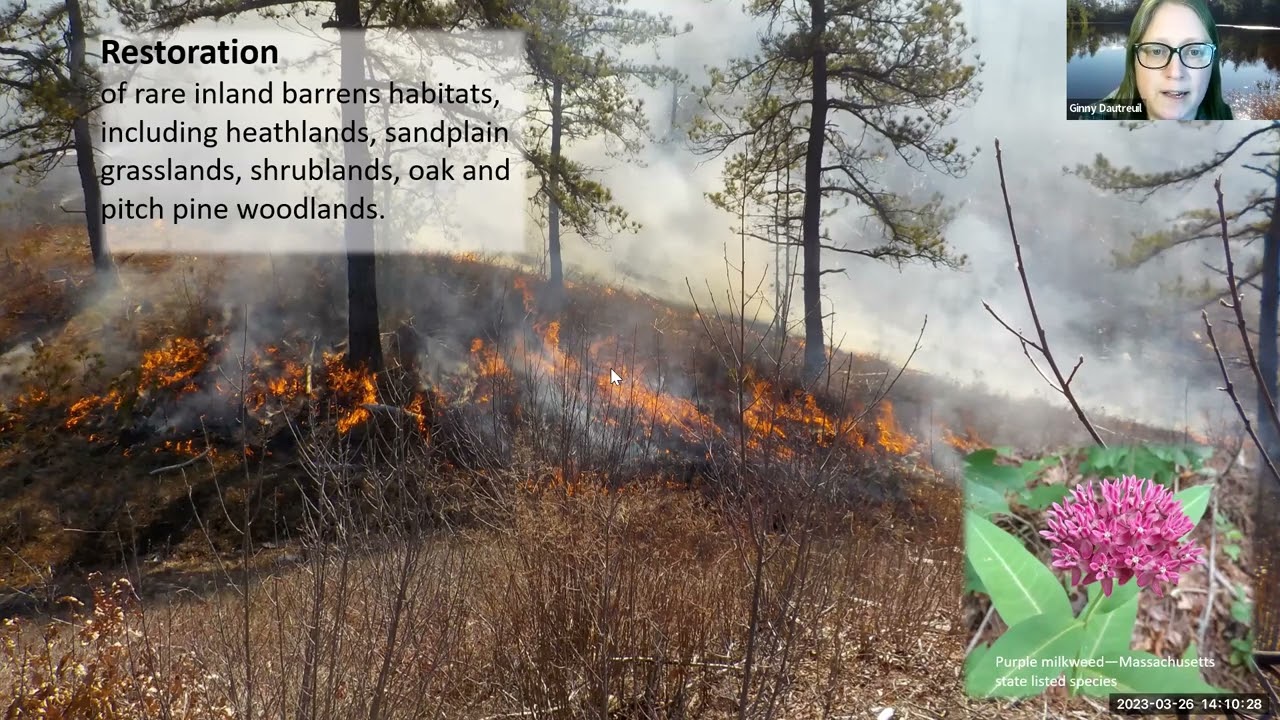The image, sourced from a presentation screen capture, conveys a detailed scene of ecological restoration. It prominently features a controlled wildfire burning through the base of several tall trees in a wooded, hilly area. The ground, covered in brownish grass and leaves, is dotted with pockets of fire and thick smoke, creating a mix of light and dark gray hues in the background. In the foreground, there is a distinctive purple milkweed flower with green leaves, identified as a Massachusetts state-listed species. The title "Restoration" is boldly printed in the upper left corner, followed by a subtitle that reads, "of rare inland barrens habitats, including heathlands, sandplain, grasslands, shrublands, oak, and pitch pine woodlands." Additionally, the image includes overlay elements: a small window in the top right corner features a white woman with glasses and straight brown hair, named Ginny Daltreau, speaking, likely about the importance of controlled fires for ecological resiliency. The date and timestamp "3-26-23, 14-10-26" appear faintly at the bottom right. A superimposed image of the purple milkweed is also positioned in this corner. This snapshot vividly portrays the transformative power of fire in habitat restoration efforts.